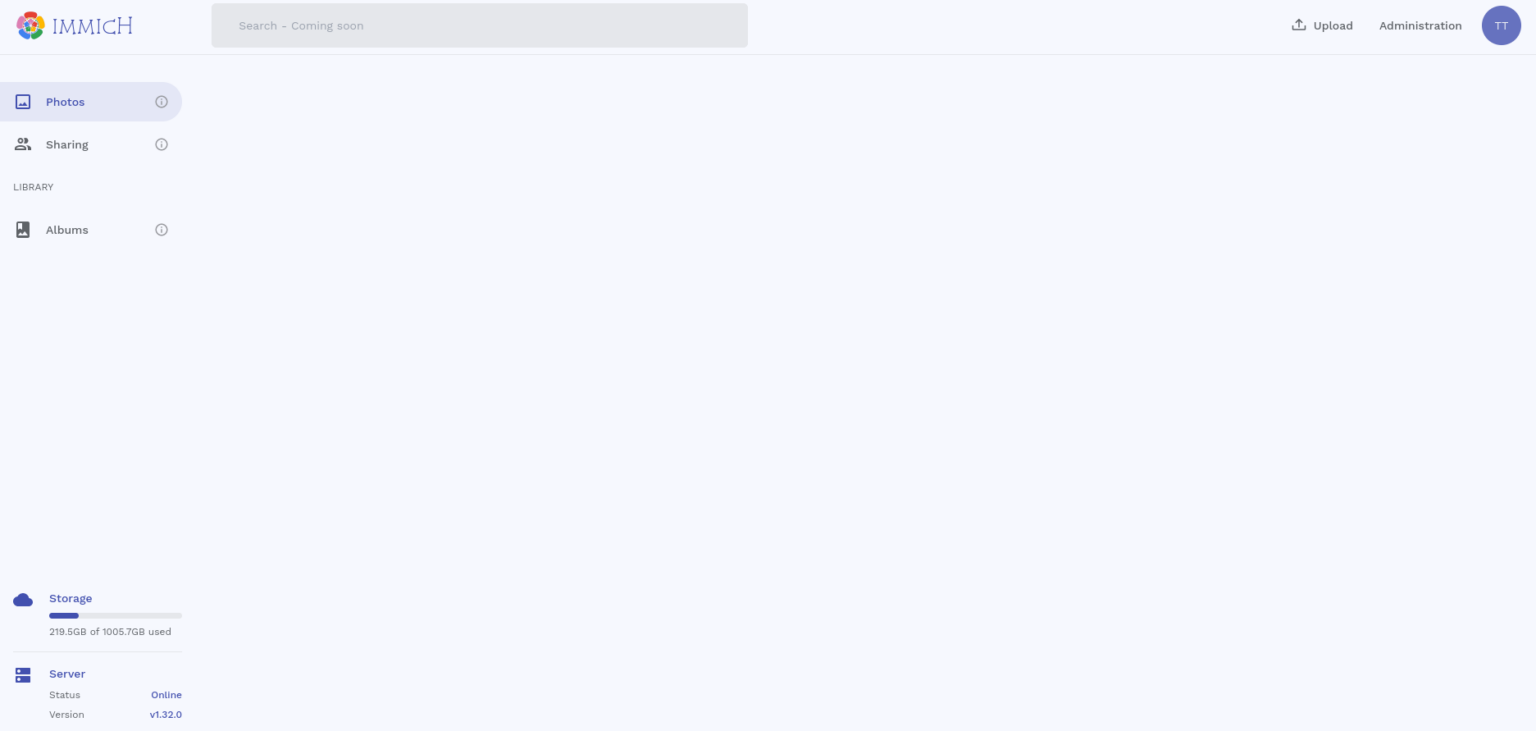This image showcases a webpage featuring an application for photo management and sharing, exemplifying a user-friendly interface designed for efficient organization and storage of images. 

In the upper left corner, a circular icon featuring a red, gold, and green color scheme catches the eye, signifying perhaps the app's logo or a brand identifier. Directly to the right of this icon, the application's name "IMMICH" is displayed prominently in bold letters. Adjacent to the app name, a light gray search bar is available for users to quickly locate specific photos or albums within the platform.

In the upper right corner, the interface includes several key functional buttons: an upload button for adding new photos, an administration button for managing settings, and a user icon, likely for accessing account details and preferences.

Underneath the logo on the left-hand side, a navigation menu organizes the app's features into easily accessible tabs. These tabs include "Photos" for viewing individual images, "Sharing" for managing shared media, and "Library" for accessing the app’s broader collection of photos and albums. Within the library section, a specific tab for "Albums" allows users to navigate through grouped collections of images.

In the bottom left corner of the interface, the storage section displays vital information about space usage, including used storage and maximum available capacity, ensuring users can manage their photo collections without exceeding limits.

Overall, the app offers a comprehensive and visually organized approach to photo management and sharing, supporting various user needs from storage to administration.